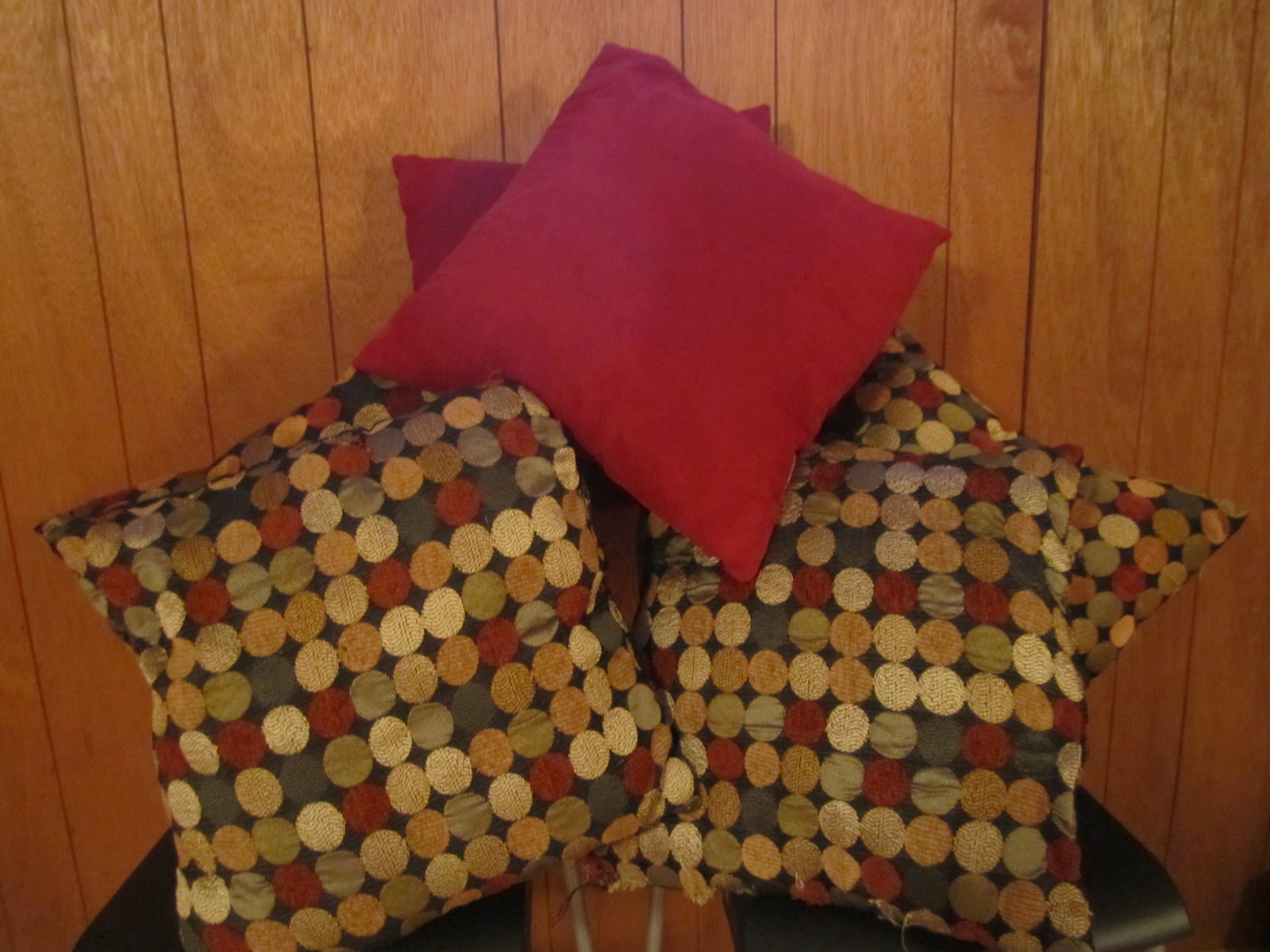The image features a set of square throw pillows meticulously arranged against a vertical wood-paneled wall that spans the height of the picture. The paneling comprises approximately 15 alternating broad and slim wooden slats, lending a rustic, retro ambiance reminiscent of the 70s and 80s. At the forefront, two vibrant red throw pillows stand out; the topmost red pillow rests diagonally, almost askew, with a matching red pillow partially visible behind it. Below these, a pair of larger pillows, each adorned with a lively polka dot pattern, blend hues of gold, white, red, green, orange, maroon, light green, dark blue, and peach in a random yet harmonious order. These larger pillows rest on the black seat pads of two kitchen-style chairs, of which only the tops are visible, hinting at their functional role in the background. The precise arrangement and vivid colors create a striking visual against the vintage wooden backdrop.